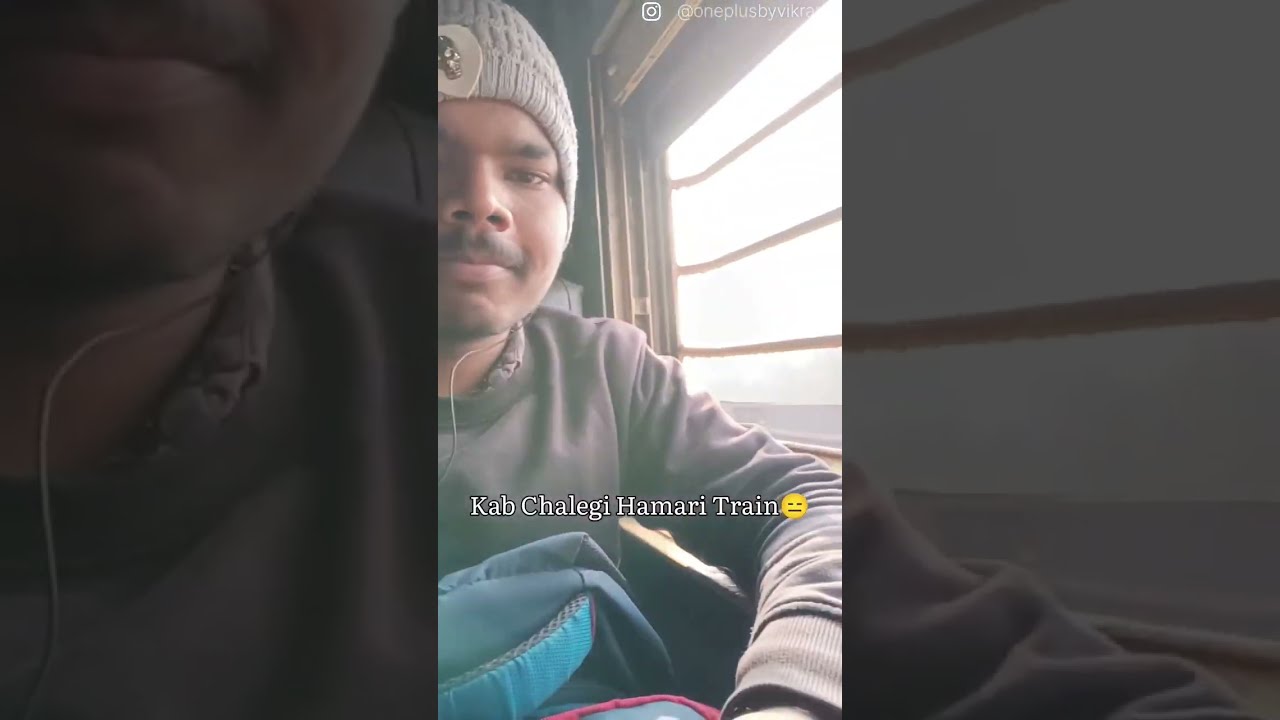This is a color photograph in portrait orientation, resembling a cell phone selfie. The photo is inset within a larger, darkened background image, which is an enlarged portion of the same photograph displayed in landscape orientation. In the brightly lit center of the image, a young, dark-skinned man, appearing to be around 20 years old, is seated inside a train car near a window. He is facing the camera with a slight, closed-mouth smile and is wearing a gray beanie with a small symbol on it, a beige sweater, and earphones with a visible wire. In his lap, he holds what seems to be some luggage, covered in blue and red fabric. The bright sunlight streams through the train window beside him, illuminating his relaxed expression. Across the bottom third of the image, the text "CAB CHELEGE HAMARI TRAIN" is displayed along with a smiley emoji. The upper part of the image contains an Instagram symbol and a user handle. The entire composition uses a representational photographic realism style, focusing on the individual’s content and serene presence during his journey on the train.